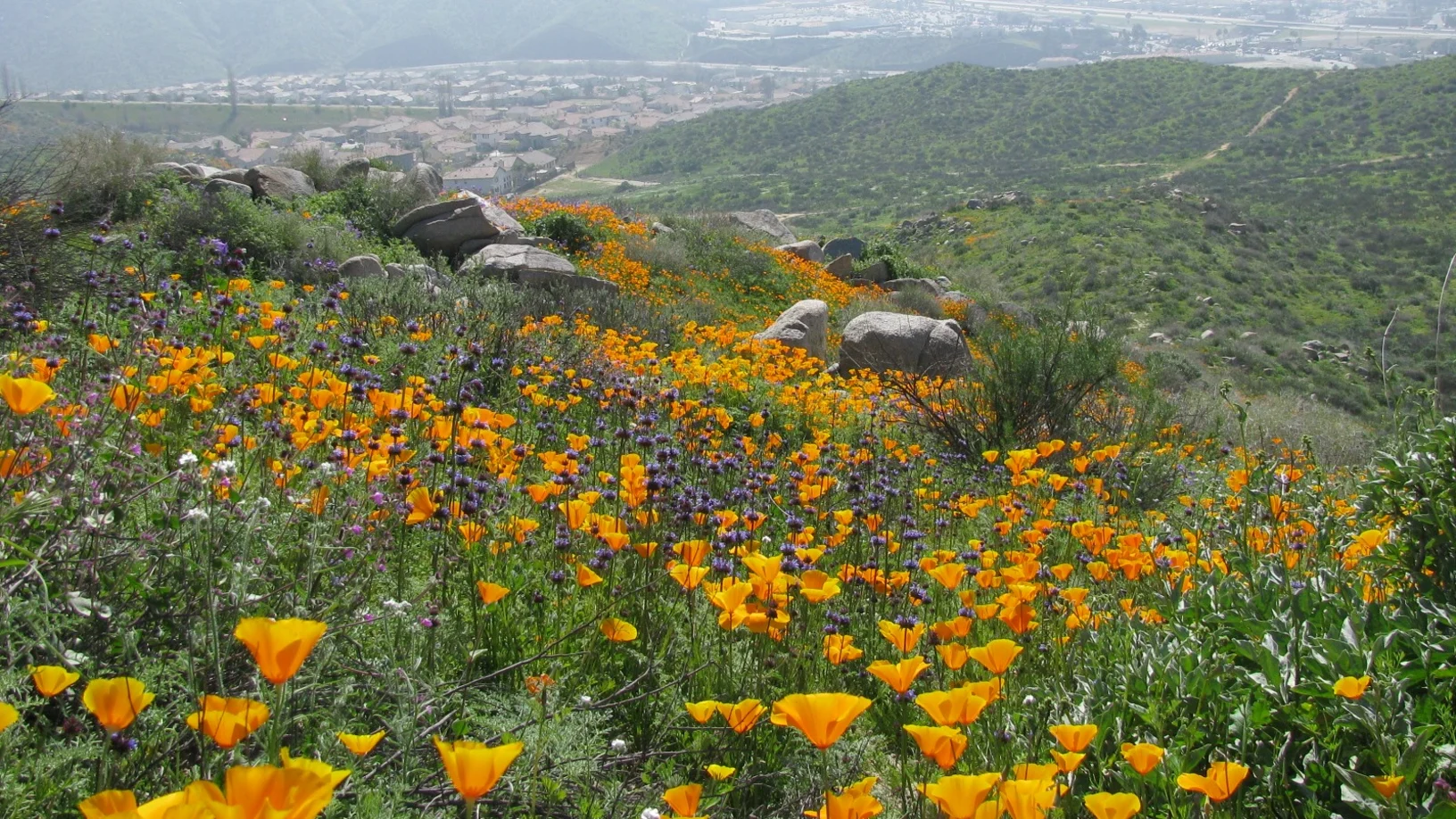This image captures a picturesque and vibrant field of wildflowers on a hillside during midday in springtime. The foreground is dominated by bright orange California poppies, complemented by a variety of smaller purple flowers and subtle white blossoms scattered throughout. The middle and bottom of the frame are adorned with these flowers, which extend and bloom their way up toward the upper middle part of the photo. Among the flowers are patches of taller grass, little bushes, and numerous rocks, creating natural pathways that add texture to the landscape.

The photo's background features a mix of more rocks and taller grass, with a hint of fog creating a soft, distant atmosphere. Far in the background, approximately half a mile away, a suburban housing development becomes visible, set against a backdrop of additional hills. On the right side of the image, there is a glimpse of an interstate highway in the top corner, further emphasizing the juxtaposition of serene nature and suburban sprawl. The overall scene offers a very pleasant and serene view, highlighting the beauty of a wildflower field in full bloom.